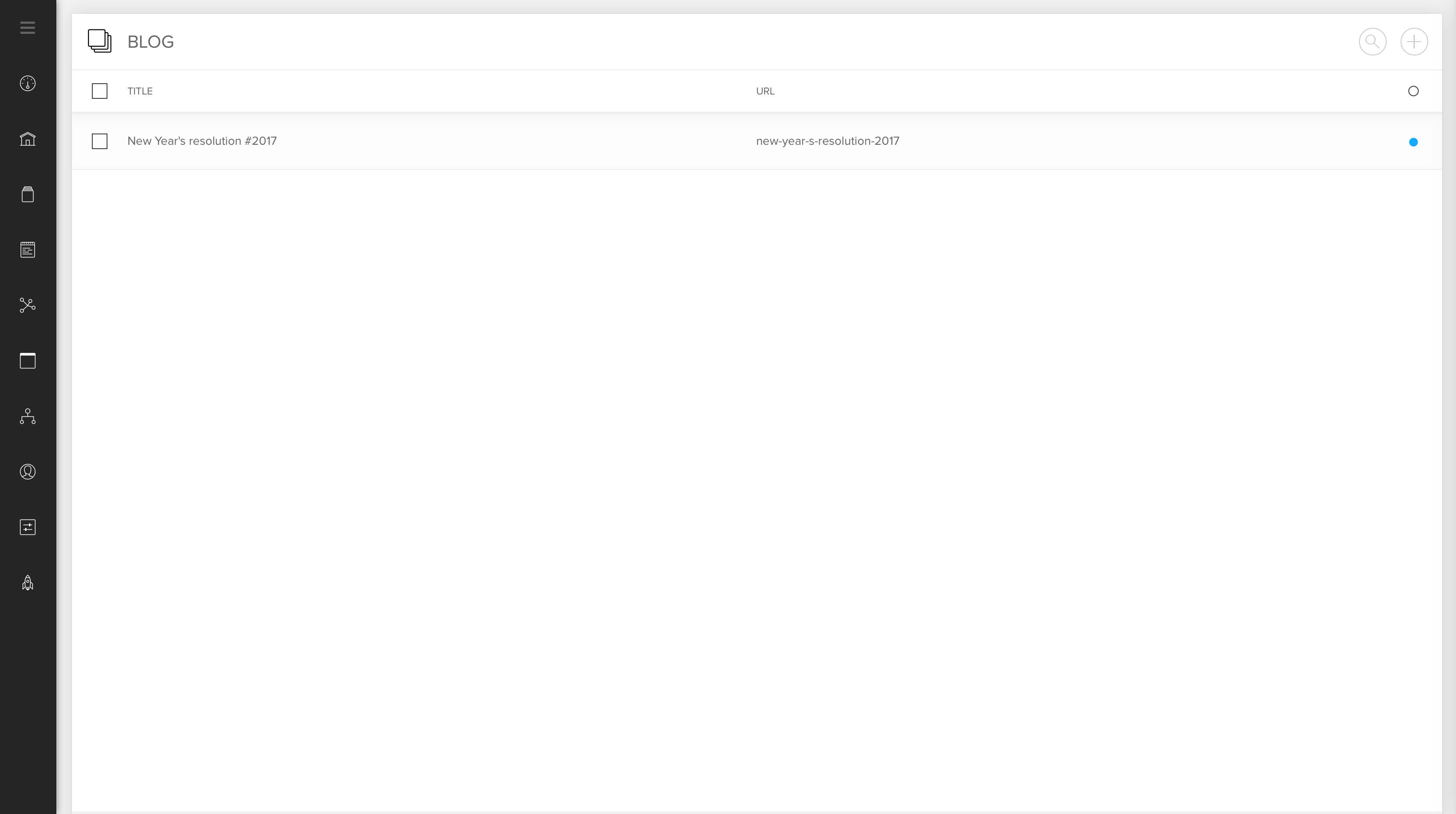The image depicts a computer screen in landscape orientation with a light gray border along the top and right-hand side. A thick gray line runs horizontally across the top and vertically along the right edge. On the left side of the screen, a thick black bar displays ten white icons in a vertical sequence, though they are too small to identify. The main view within the gray-outlined rectangle shows a header labeled "Blog" with a small icon resembling screens or pages beside it. Below this, there is a field labeled "Title" followed by a pale gray bar, which appears to include text beginning with "New Year's Resolutions," though the year is indiscernible. The body section beneath these fields is blank, indicating that it is likely a template for a blog post. To the right of the header, there are two circular icons: one with a magnifying glass representing a search function and the other with a plus sign likely indicating an option to add content. The bottom of the screen features a very thin gray border, contrasting with the thicker borders on the top and sides.